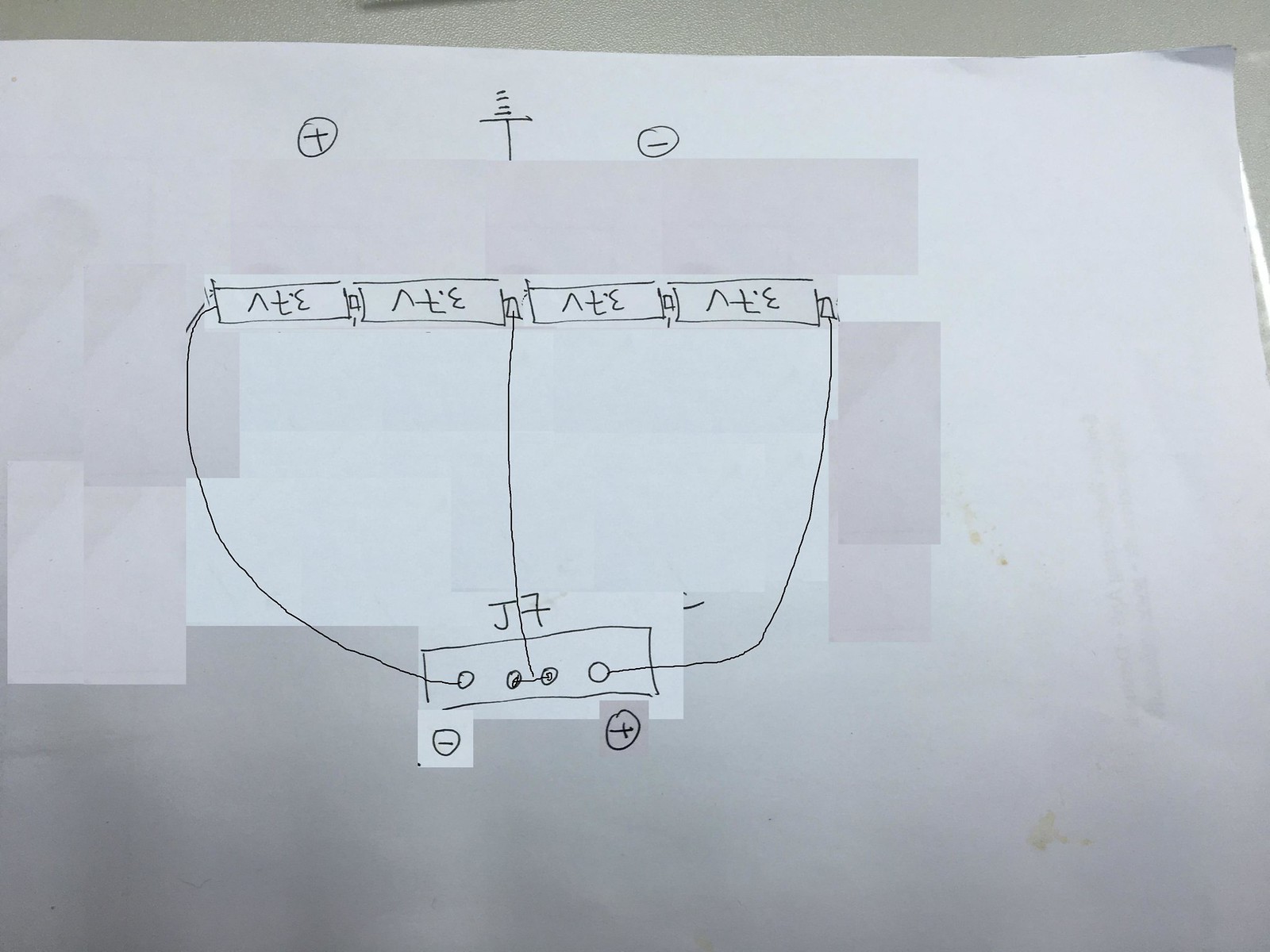In the image, a gray surface serves as the background. On this surface lies a white, unlined sheet of paper with noticeable food stains clustered on the right side, presenting a brownish hue. The top of the page features a hand-drawn ink pen sketch of a circle with the letter "T" at its center. Adjacent to this circle, on the right, is another "T" overshadowed by four small vertical lines. Further to the right is yet another circle containing a single horizontal line.

Below this, there is a light pink rectangle, under which are four smaller rectangles resembling batteries. Each battery-like shape is characterized by an extension on the right side, an inverted arrow, a lowercase "t," and a capital "E." These elements are interconnected by two curved lines originating from the right side, extending downward to a larger rectangle at the bottom, which is detailed with four circles on its lower edge. This larger rectangle features a "J," a "7," and a line connecting it back to the upper "batteries." 

Additionally, there is a circle intersected by a line, positioned beside a white square on the lower segment of the page. To the right of this configuration, a pink square is visible, adorned with a circle that contains a lowercase "t."